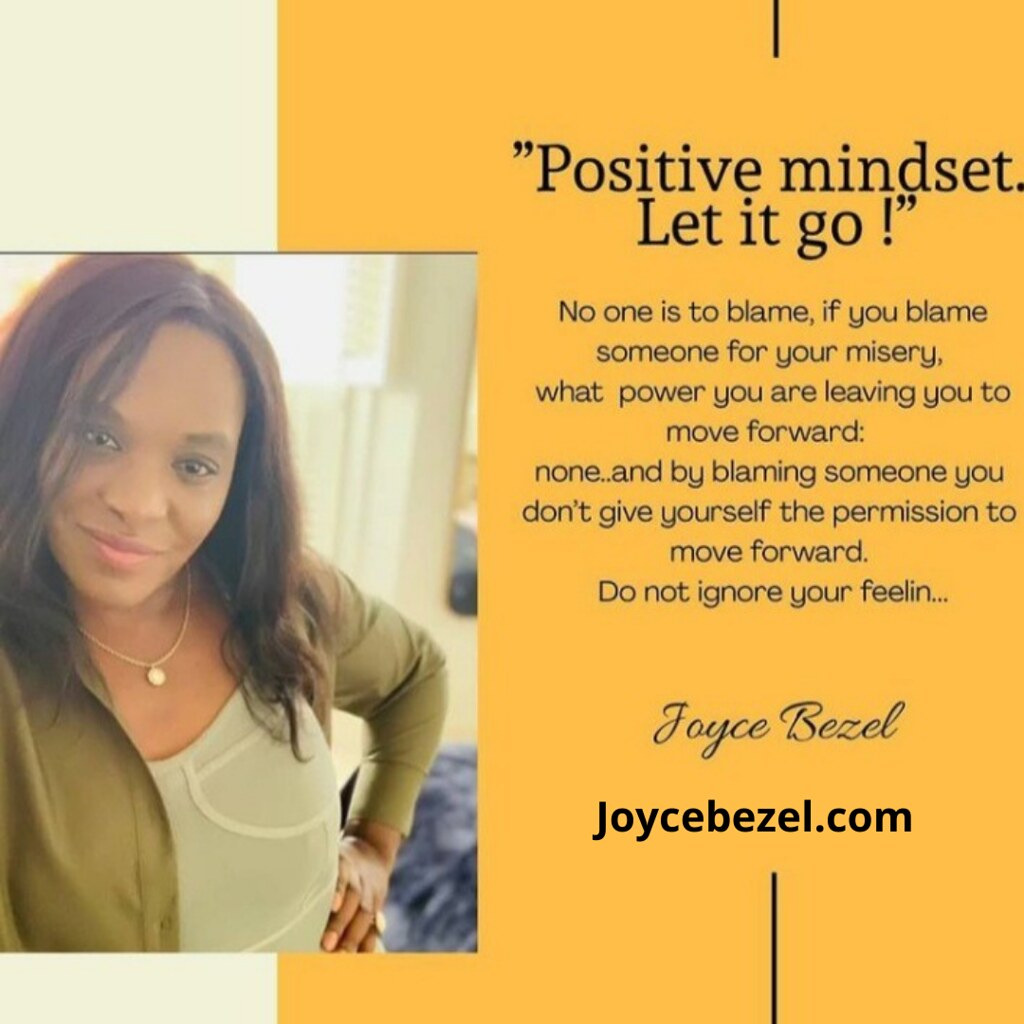The poster advertises a website for Joyce Beasle, who appears to be a motivational speaker or life coach. The square image features an orange background with a lighter orange strip along the left side. On the left side of the poster, there's a picture of a woman, presumably Joyce Beasle, standing with her hand on her hip, angled slightly with her head tilted. She exudes a professional demeanor, dressed in a green jacket over a lighter green shirt and a stylish necklace. Her long brown hair is neatly styled, adding to her polished appearance.

At the top right, the poster displays the title and quote in bold black letters: "Positive Mindset, Let It Go." Below the quote, a more detailed message extends advice about the drawbacks of blaming others for one's misery and the importance of taking responsibility to move forward. The text reads, "No one to blame. If you blame someone for your misery, what power are you leaving you to move forward? None. By blaming someone, you don't give yourself permission to move forward. Do not ignore your feeling."

Joyce Beasle's name and her website, JoyceBeasle.com, are prominently mentioned, reinforcing her brand as a figure focused on personal growth and positive mindset coaching. The background also incorporates accents of yellow and white, contributing to an overall uplifting and encouraging aesthetic.